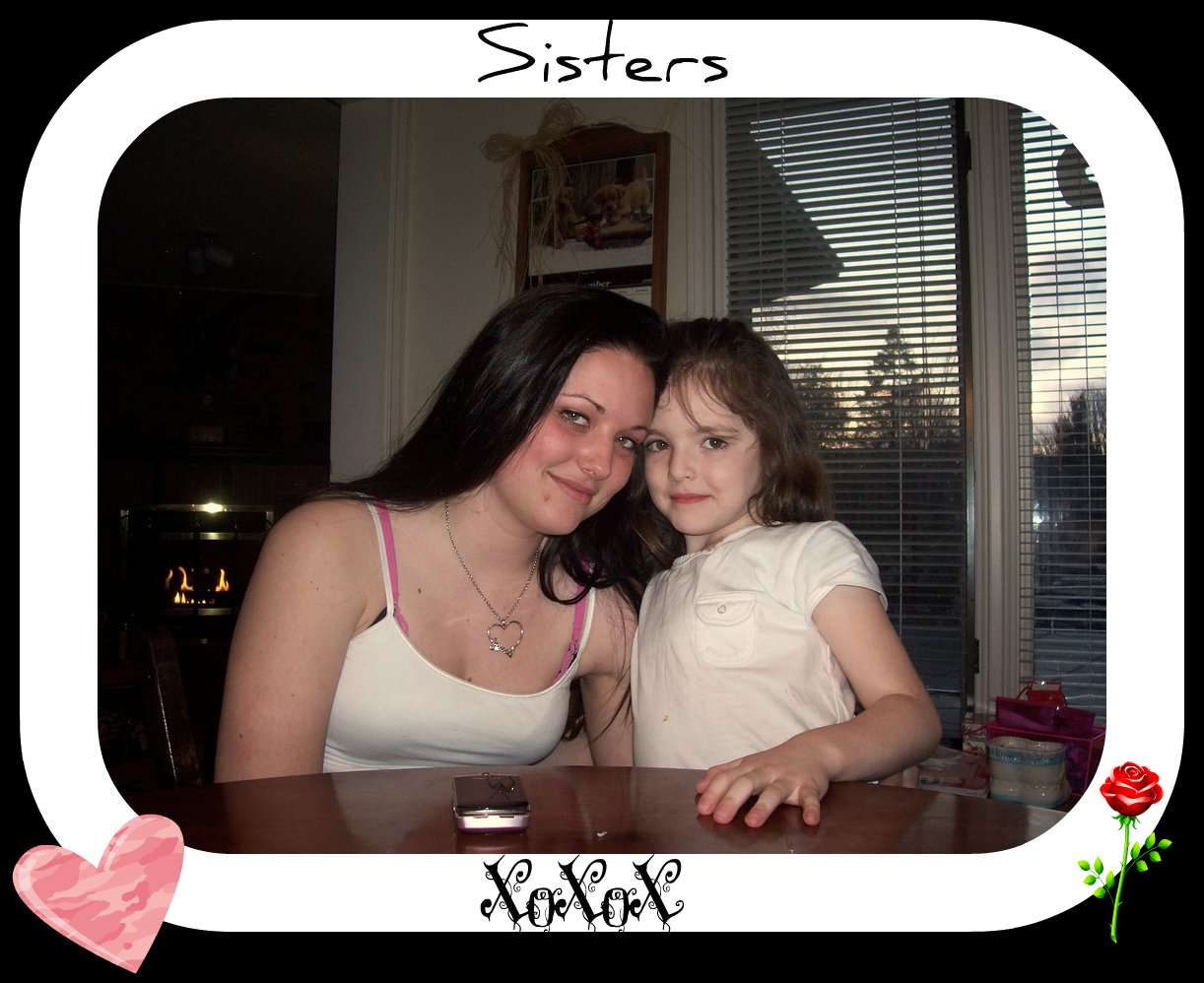In the image, a teenage girl with long dark brown hair, wearing a spaghetti strap blouse with visible pink straps underneath, is sitting and leaning slightly towards the center. She is adorned with a heart necklace and has her head touching that of a younger girl. The younger girl, who has lighter brown hair and is standing, is wearing a white shirt and has her hand resting on a table in front of them, next to a phone positioned to the left. Both girls are smiling warmly at the camera.

The background features a wall with a calendar, a fireplace to the left behind the older girl, and tall windows with shades to the right. The photograph is framed with a rounded white border. At the top of the border, the word "sisters" is penned in what seems to be magic marker or pen. The bottom of the border has "XOXOX" inscribed, along with a pink heart in the bottom left corner and a red rose in the bottom right corner.